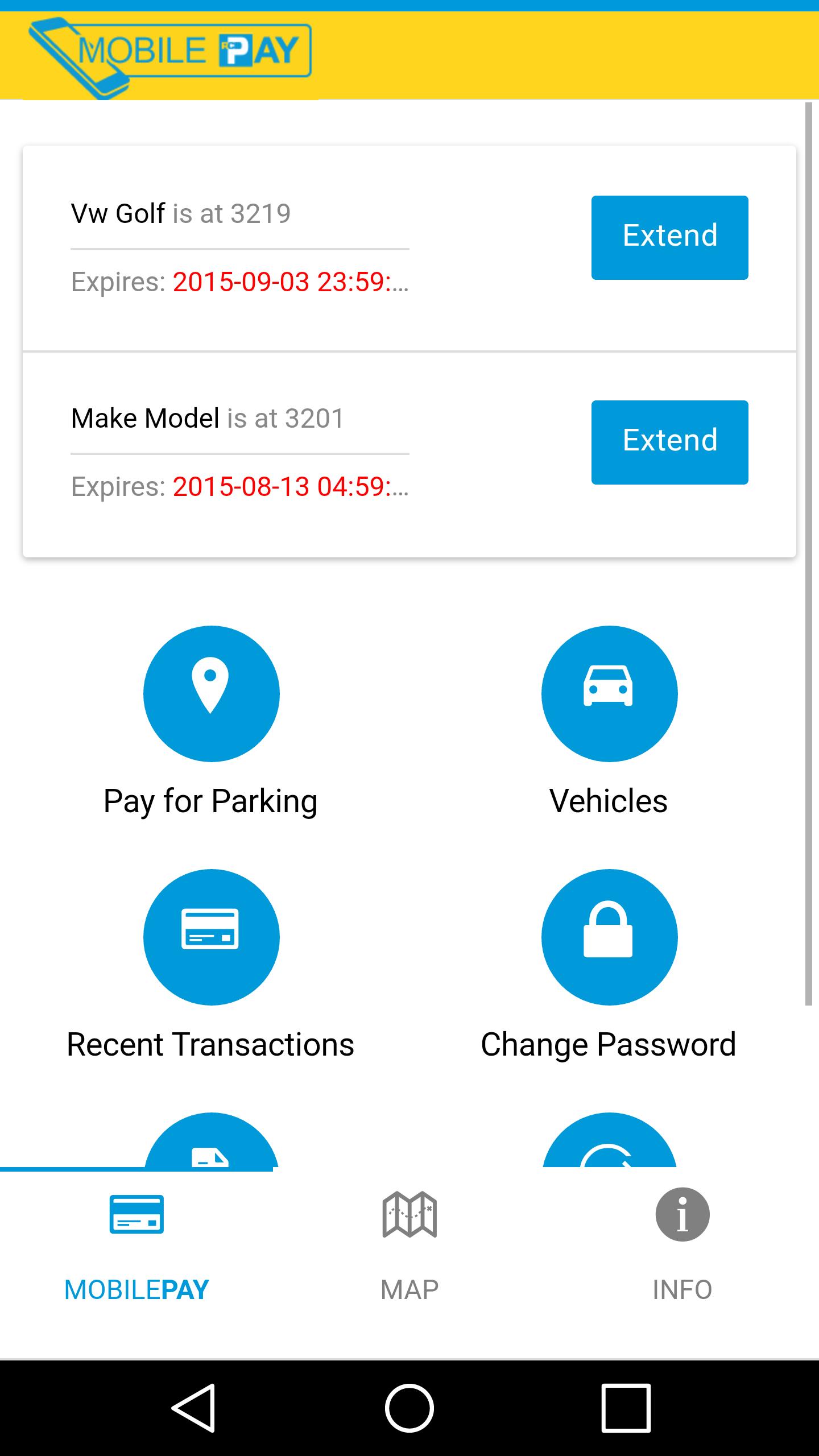**Detailed Caption:**

This image is a screenshot of an application interface, likely viewed on an Android device, as inferred from the three navigation symbols present at the bottom of the screen—a triangle pointing left, a circle in the center, and a square on the right. The application in view is "MobilePay," evident from its logo at the top, which consists of the text "MobilePay" in blue and yellow alongside an icon of a diagonally-oriented phone.

The app's color scheme primarily features white and blue, with yellow highlights used sparingly on the top bar. At the interface's top section, there are two notable entries labeled "VW Golf" and "Make Model," each accompanied by an "extend" button that presumably allows the user to elongate some form of service or entry.

Below these entries are six buttons arranged in two vertical rows of three. However, the bottom two buttons are partially obscured, revealing only their upper halves. The visible button labels, read from left to right, are as follows:
1. "Pay for parking"
2. "Vehicles"
3. "Recent transactions"
4. "Change password"

The partially visible labels of the bottom two buttons remain unidentified due to the cutoff.

At the bottom of the interface, there is a navigation bar with three options: "MobilePay," "Map," and "Info." The "MobilePay" option is currently selected, indicating the active view of the screenshot. The app seems to offer functionalities related to parking payments, vehicle management, transaction history, and password changes, suggesting a comprehensive utility for users managing multiple vehicles or frequent payments.